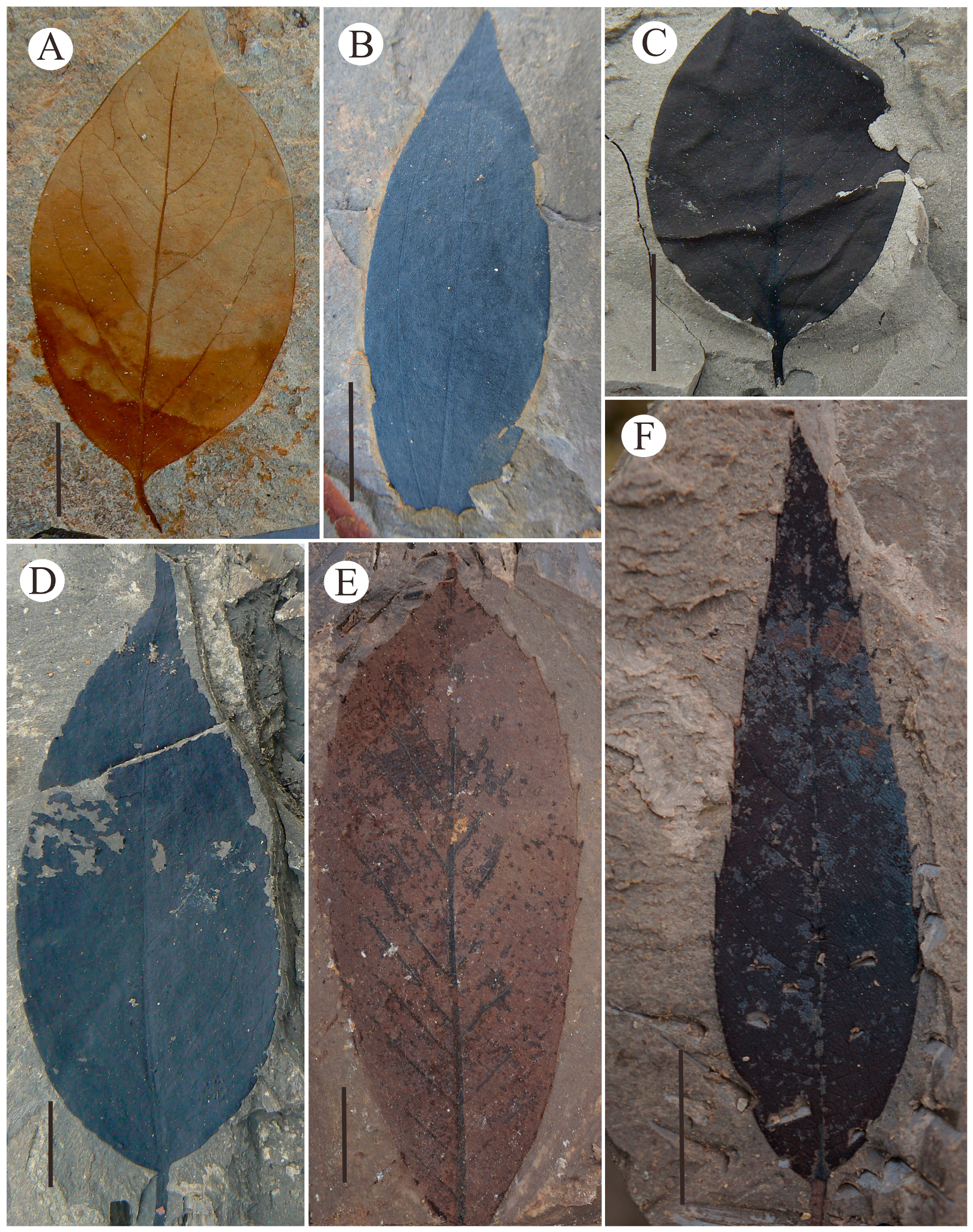The image features six distinct panels, each segmented with white outlines and showcasing a unique leaf against a stone-like background. The panels are labeled with white circles and black lettering: A, B, and C at the top, and D, E, and F at the bottom. Panel A displays an orangey-brown leaf with intricate veining. Panel B contains a blue teardrop-shaped leaf, while panel C features a somewhat deteriorating round leaf in a brown or dark gray shade, resembling a seed pod. At the bottom left, panel D shows another blue leaf similar to B but with white markings. Panel E, to the right of D, presents a salmon-colored leaf with notable veining patterned from the central stem. Finally, panel F on the bottom right depicts a tall, slim, and pointed leaf with ridge edges, appearing almost black. Each leaf appears to be painted on a textured, stone-like background, enhancing the fossilized aesthetic of the artwork.